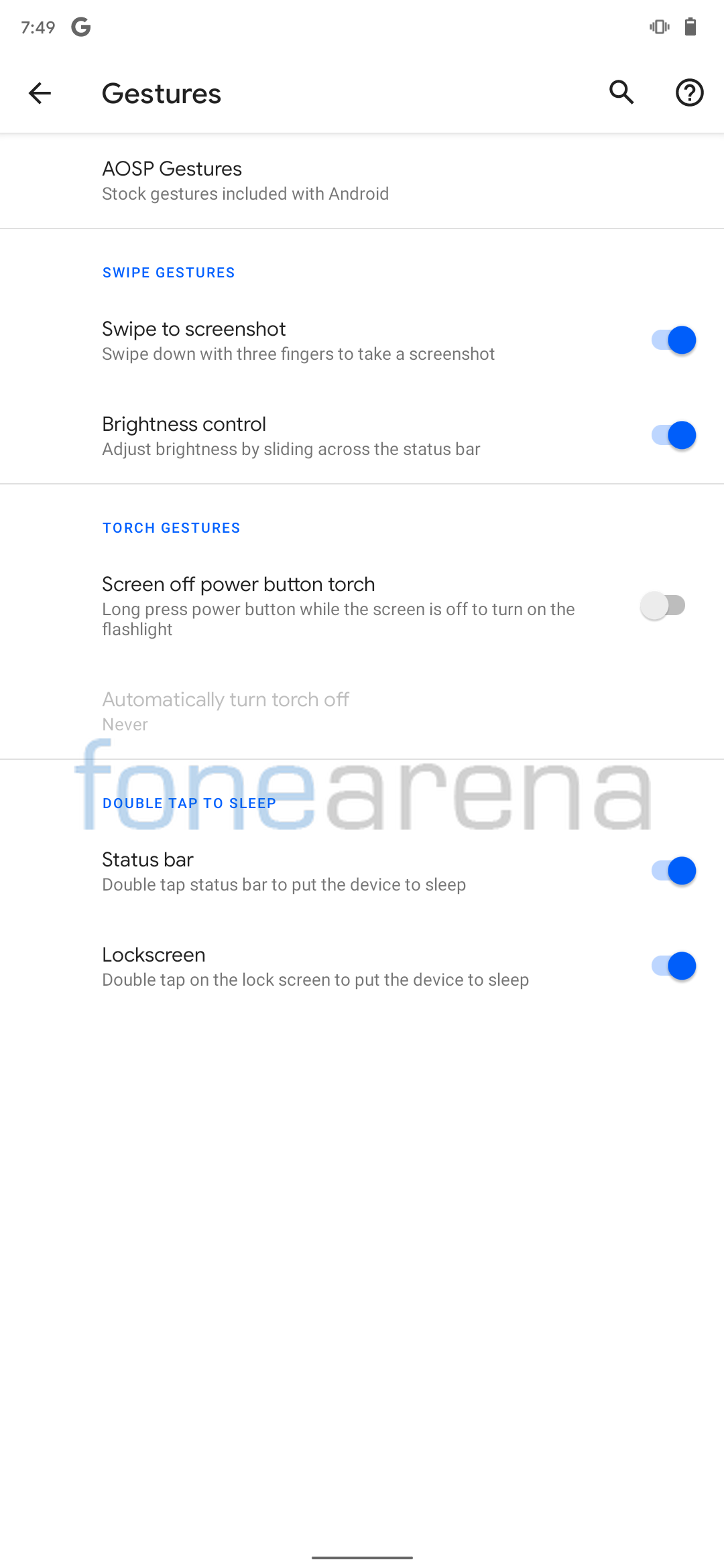This screenshot captures a webpage displaying various settings and gestures for an Android device. In the upper left-hand corner, the time is shown as 7:49, accompanied by a large grey "G" logo. On the upper right-hand side, an image of a battery is shown. Below these elements, a light grey line separates the header from the content.

The content is divided into columns and categories, starting with a section titled "A Q S P G E S T U R E S," which highlights stock gestures included with Android. Below another thin grey line, there is a section labeled "Swipe Gestures" in blue. Underneath, in black text, the instructions read: "Swipe to screenshot – swipe down with three fingers to take a screenshot." Next to this description, there is a blue button on the right-hand side.

Following that is a row labeled "Brightness Control," which details how to adjust brightness by sliding across the status bar. Again, there is a blue button to the right of this description.

Beneath another thin grey line, a section called "Torch Gestures" in blue outlines the flashlight functionality. The text describes: "Screen off power button touch – long press the power button while the screen is off to turn the flashlight off." Below this, it mentions in grey text that the torch will automatically turn off, and currently, it is set to "never." The button for this setting is in the "off" position.

Imposed over the screen is the watermark "FONEARENA," where "FONE" is in blue and "ARENA" is in grey. At the bottom, another gesture titled "Double Tap to Sleep" is featured in blue text. The descriptions below indicate that double-tapping the status bar or the lock screen will put the device to sleep. Blue toggle bars are visible on the right-hand side, indicating the settings' active states.